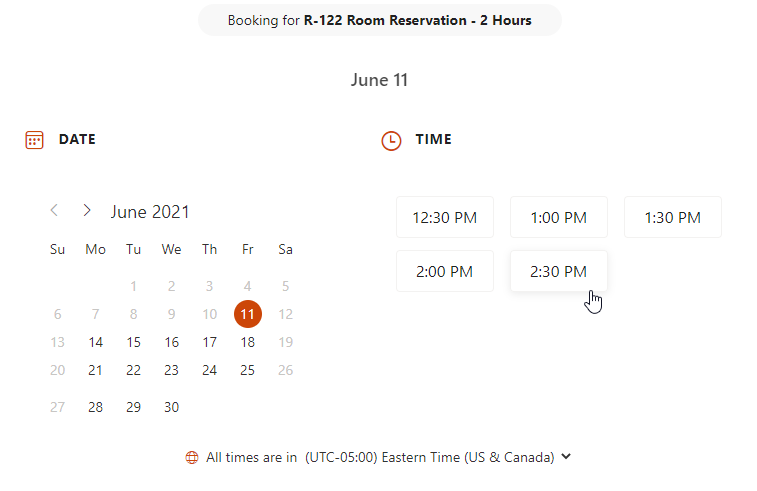The image depicts a booking website interface specifically designed for scheduling room reservations. At the top, there is a prominent gray header box displaying "Booking for R-122 Room Reservations - Two Hours" in bold black letters. Below this header, June 11th is mentioned, also in gray text.

The interface includes fields for setting the date and time of the reservation. The date is represented by a calendar icon in red, and prominently displays a calendar for June 2021, with June 11th highlighted inside a red circle. Next to the date icon, a clock icon, also in red, signifies the time setting, which is currently set to 3:00. A specific time is highlighted with a hand icon pointing to 2:30, indicating the intended start time of the booking.

Additionally, a red and white asterisk section provides important time zone information, stating "All times are in (UTC-5:00) Eastern Time (US & Canada)." This text includes a drop-down menu option for changing the time zone if necessary.

Overall, the website features clear and concise details to facilitate room booking, including specific date and time settings, time zone information, and an easy-to-read format.